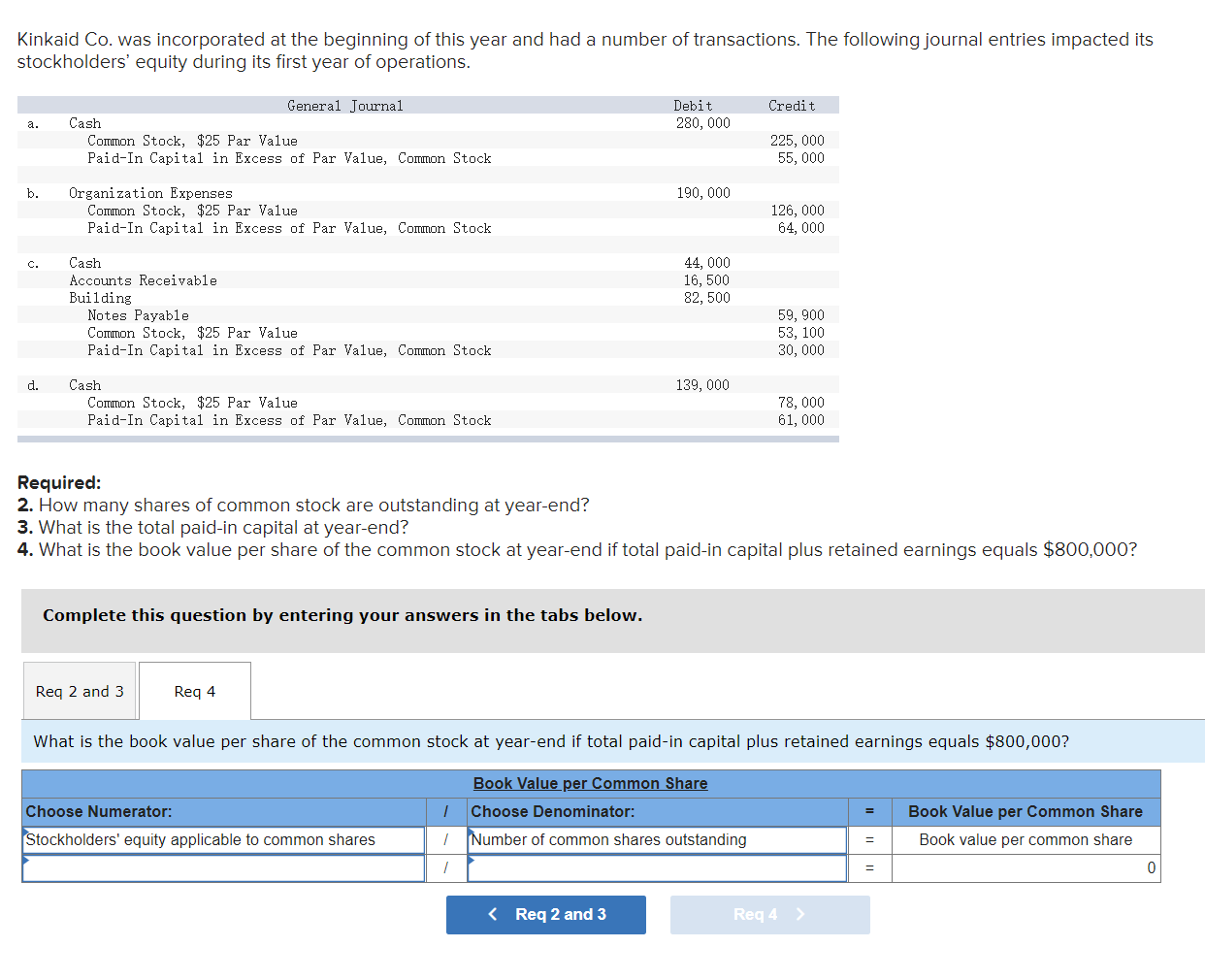The screenshot features a white background, and it begins with an informative note in black text on the upper left-hand corner stating, "Kincade Co. was incorporated at the beginning of this year and had a number of transactions. The following journal entries impacted its stockholders' equity during its first year of operations." 

Below this text, there is a section resembling an Excel spreadsheet without visible columns, titled "General Journal." To the right, there are columns designated for debits and credits, while the headings include cash, operational expenses, cash accounts receivable building, and cash again at the bottom.

On the lower left, there are several bolded, black text requirements:
1. "Required"
2. Bolded number "2": "How many shares of common stocks are outstanding at year-end?"
3. Bolded number "3": "What is the total paid-in capital at year-end?"
4. Bolded number "4": "What is the book value per share of the common stock at year-end if total paid-in capital plus retained earnings equals $800,000?"

Adjacent to these requirements is a horizontally extended gray rectangle with a bold, black text that instructs, "Complete this question by entering your answers in the tabs below."

Below the gray rectangle, there are two buttons: the left one is labeled "REQ 2 and 3" and is gray, while the right one is labeled "REQ 4" and is white. Further below, a light blue rectangle contains the question in black text, "What is the book value per share of the common stock at year-end if total paid-in capital plus retained earnings equals $800,000?" 

Subsequently, it provides column headings such as "book value per common share," "choose numerator," "choose denominator," and "book value per common share." At the very bottom, there are two additional navigation buttons, the left one having a back arrow labeled "REQ 2 and 3," and the right one with a right arrow labeled "REQ 4."